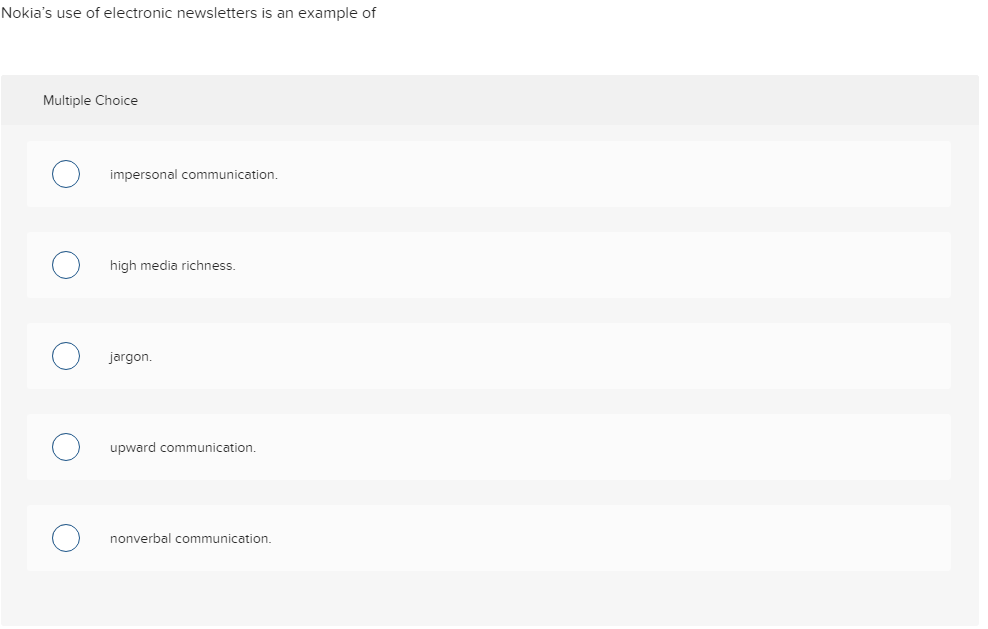The image depicts a page designed in a multiple-choice quiz format. At the top of the page, the question reads, "Nokia's use of electronic newsletters is an example of?" Beneath the question, there are five answer options: 

1. Impersonal communication
2. High media richness
3. Jargon
4. Upward communication
5. Nonverbal communication

Each answer option is enclosed in a text box with a white background and black text. Adjacent to each option is a circle with a white center and a blue border, presumably to mark the selection of an answer. The background for the entire quiz section is a light gray, providing a slight contrast to the white text boxes. This setup resembles an online quiz interface where users can click to select their response.